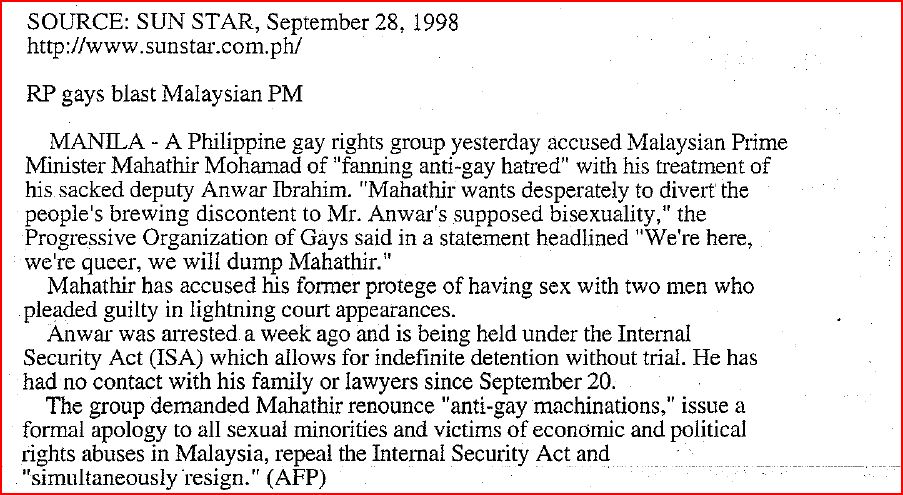This image is a screenshot resembling a newspaper article from Sunstar, dated September 28, 1998. The predominantly black, white, and red text details a story headlined "RP, Gays Blast Malaysian PM." The article reports on a Philippine gay rights group accusing Malaysian Prime Minister Mahathir Mohamad of inciting anti-gay sentiments through his treatment of his former deputy, Anwar Ibrahim. It mentions that Mahathir is allegedly using Anwar's supposed bisexuality to distract from public discontent. The group's statement, highlighted with the bold headline "We're here, we're queer, we'll dump Mahathir," demands the Prime Minister renounce anti-gay actions, formally apologize to sexual minorities and victims of broader rights abuses in Malaysia, repeal the Internal Security Act, and resign simultaneously. Anwar, accused of consensual sex with two men who faced swift court proceedings, has been detained under the Internal Security Act without contact with his family or legal representation since September 20. The article contains references to additional web links and thorough details on the political tension underlying the cited events.